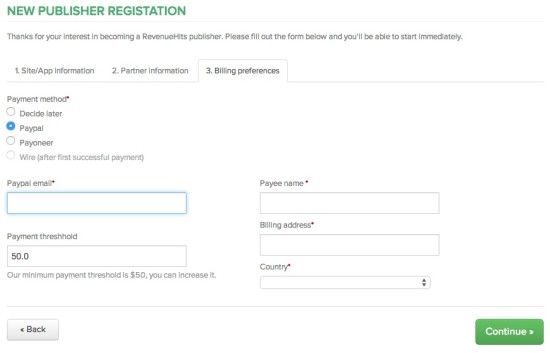The screenshot displays a registration interface for a subscription service, featuring a clean, white background. At the top, "New Publisher Registration" is prominently shown in medium green text. Below, dark gray body text thanks users for their interest in becoming a Revenue Hits publisher and invites them to fill out the form to start immediately.

The form is divided into three tabs: "Site/App Information," "Partner Information," and "Billing Preferences," with the "Billing Preferences" tab currently active. This tab includes a section titled "Payment Method" with four radio button options: "Decide Later," "PayPal," "Payoneer," and "Wire (after first successful payment)." The "PayPal" option is selected by default.

Underneath the payment method section, there are additional fields: a text box for entering the PayPal email address, fields for the payee's name and billing address, and a dropdown list for selecting the country.

To the left, there is a section for "Payment Threshold" set to $50, with a note clarifying that the minimum payment threshold is $50, but it can be increased.

At the bottom of the interface, a navigation bar includes two buttons: a gray "Back" button with black text and a left-pointing arrow, and a green "Continue" button with white text and a right-pointing arrow.